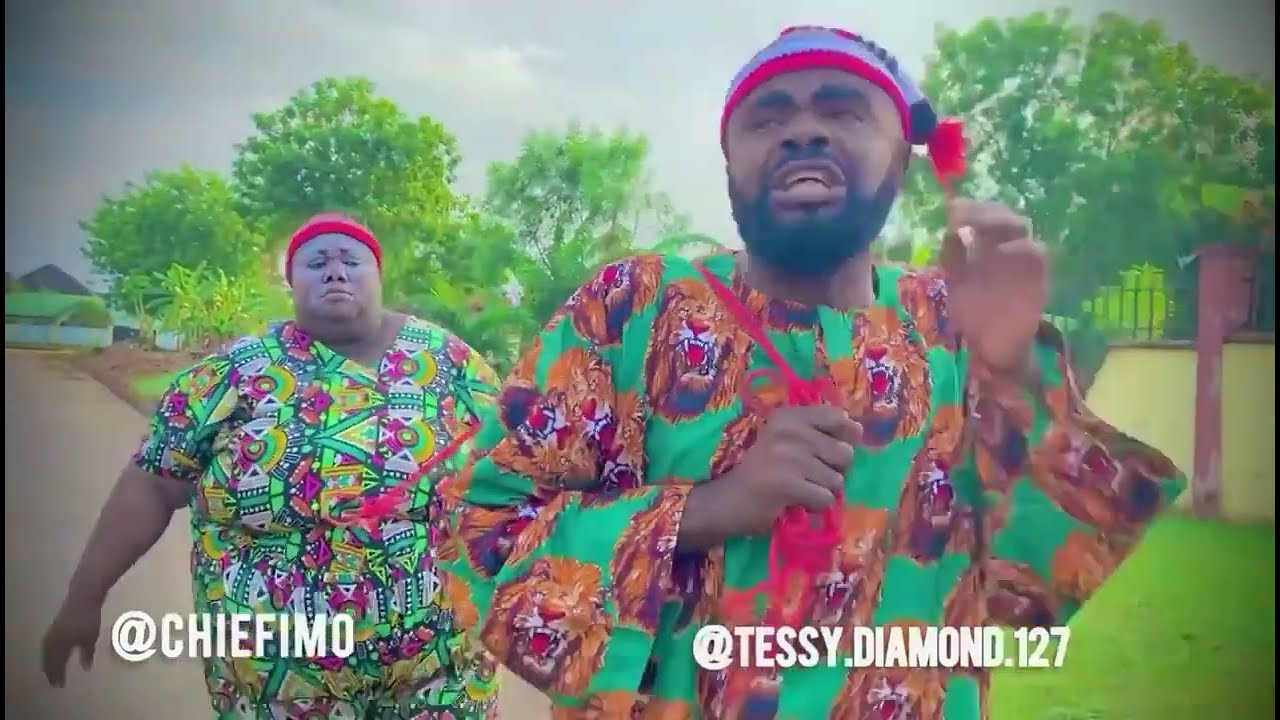In this image, we see two African-American individuals wearing traditional African attire, seemingly captured from a YouTube thumbnail or a screen grab from a video. The man on the right, who is heavyset and bald, is dressed in a vibrant lime green shirt adorned with images of roaring lions and intricate African patterns. He wears a winter hat with a red band and a red tassel. His arms are raised as if he is running, and his expression shows a mix of determination and fatigue.

Next to him is a woman in a multicolored African dress with geometric patterns. She appears to be slightly behind him, also in motion, although not as fast. Adorned with a red headscarf, she too has a concerned expression on her face. The background features stylized trees, fences, and houses, giving the scene a washed-out, slightly colorful manipulative look. Below each individual, social media handles are displayed: "@ChiefIMO" for the man and "@TessieDiamond127" for the woman. The overall setting suggests they are on a dusty road, possibly in an African village, with a sense of urgency and movement conveyed through their postures and expressions.